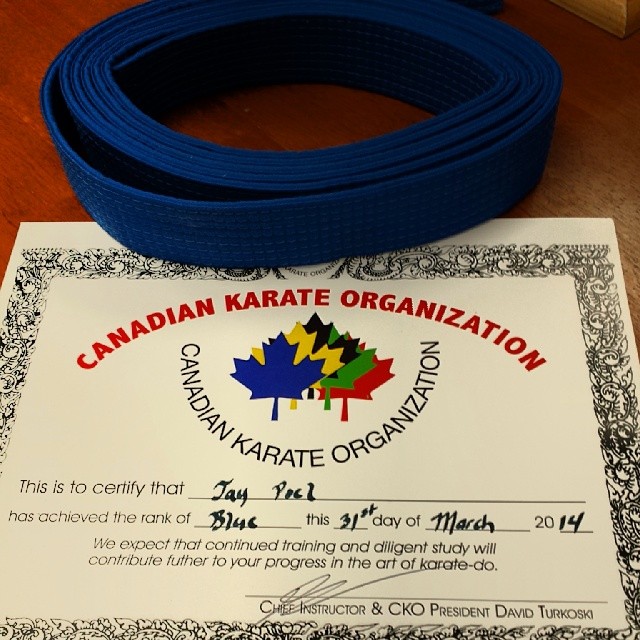The image captures a certificate and a blue belt displayed on a wooden table. The certificate announces the achievement of Jay Paul, who has earned the rank of blue as of March 31, 2014, under the auspices of the Canadian Karate Organization. The certificate is adorned with a black floral border and prominently features the organization's name in red, along with an arched text in blue shaped like a semi-circle. The logo includes maple leaves in various belt colors—blue, yellow, black, green, and red—stacked at an angle. It concludes with an encouraging note for continued training and is signed by Chief Instructor and CKO President, David Turkoski. The blue belt is neatly rolled up and placed adjacent to the certificate, ready to be presented to its recipient.